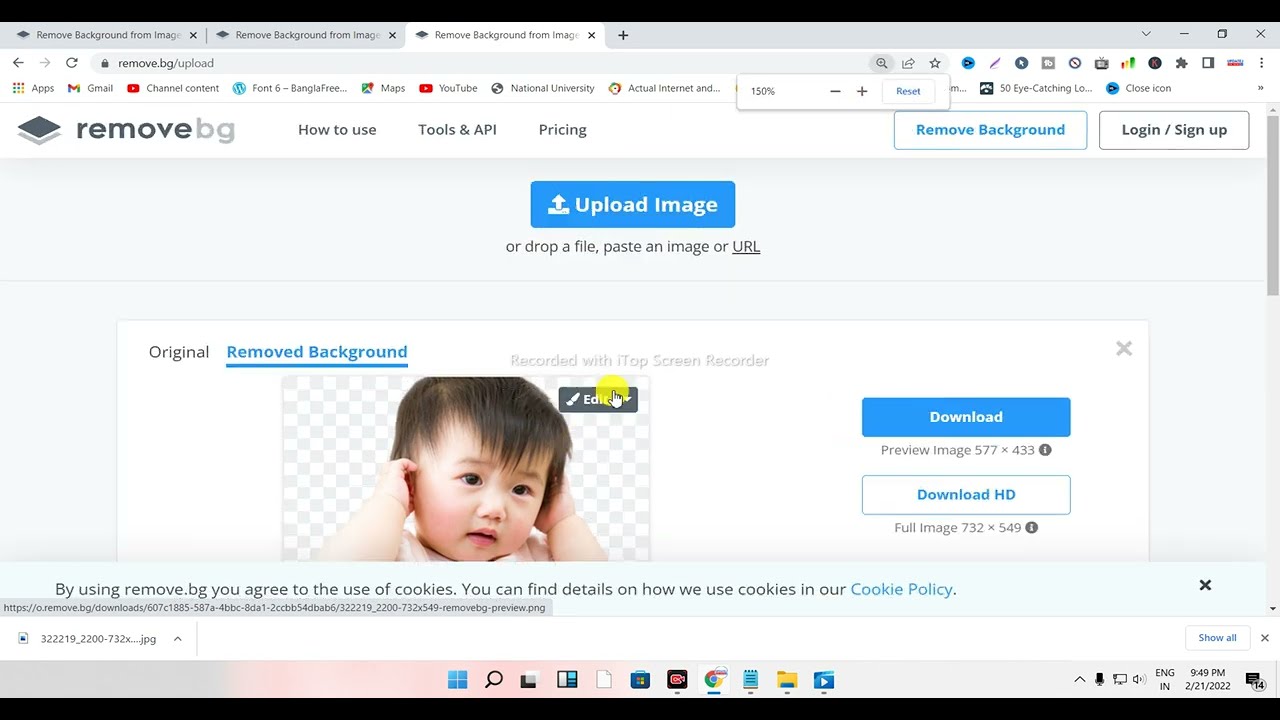The screenshot captures the interface of a web page displayed on a computer monitor running Windows 11, with visible toolbars, taskbars, and application icons like Google Chrome and Windows Media Player at the top. The website, identified by its URL as Remove.bg, is showcased in the third browser tab alongside the white strip header with the text "Remove BG" in gray font. Adjacent to the header text are navigation options: "How to Use," "Tools and API," and "Pricing," followed by a login area and a blue rectangle with "Remove Background."

Below the header, the web page, set against a gray background, prominently features a blue rectangular button labeled "Upload Image." Directly beneath this button, there is a photograph of a toddler, specifically an Asian baby's head, with the background successfully removed as indicated by the surrounding options showing "Original" and "Removed Background." To the right of the baby’s image, there are two buttons: a blue one labeled "Download" and a white one labeled "Download HD." The entire presentation is framed by thin black rectangles at the top and bottom, suggesting it's a wide rectangular image.